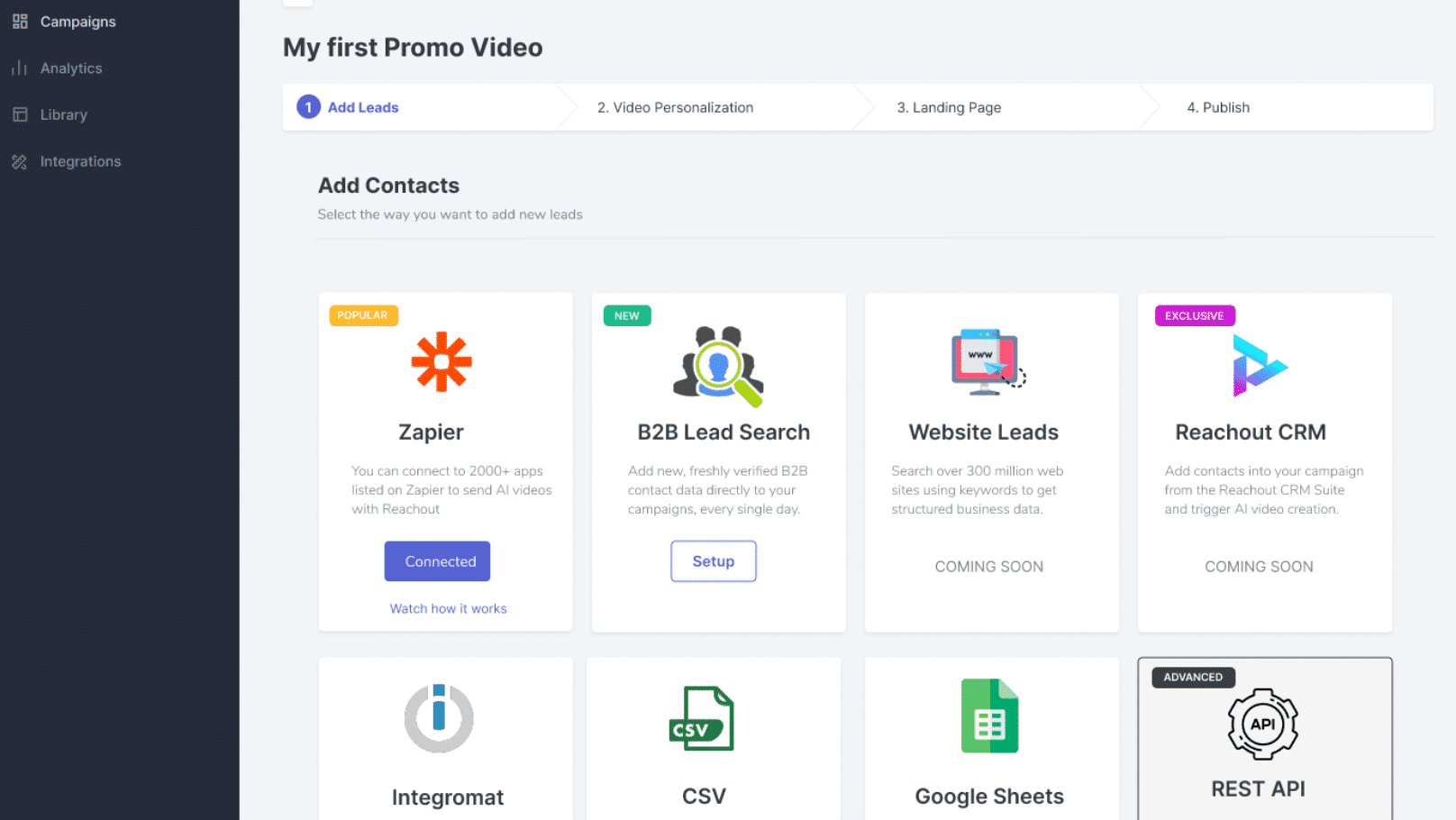The image depicts the interface of a lead-generation application set against a light blue background. On the left, there is a dark blue vertical sidebar with menu options written in a lighter blue: "Campaigns," "Analytics," "Library," and "Integrations." 

In the main body of the interface, the top section is titled "My First Promo Video." Below this title, the lead generation process is outlined in three steps:

1. Add Leads
2. Video Personalization
3. Landing Page

Directly beneath these steps, there is an instruction that reads, "Add Contacts. Select the way you want to add new leads."

The interface displays eight different options for adding leads, arranged in two rows of four boxes each:
- Upper Left: **Zapier** - Connect to 2,000+ apps listed on Zapier to send AI videos with ReachOut.
- Upper Center Left: **B2B Lead Search**
- Upper Center Right: **Website Leads**
- Upper Right: **ReachOut CRM**

- Lower Left: **Intergromit**
- Lower Center Left: **CSV**
- Lower Center Right: **Google Sheets**
- Lower Right: **REST API**

This application is designed to facilitate the process of adding and managing leads through various integrations and tools.